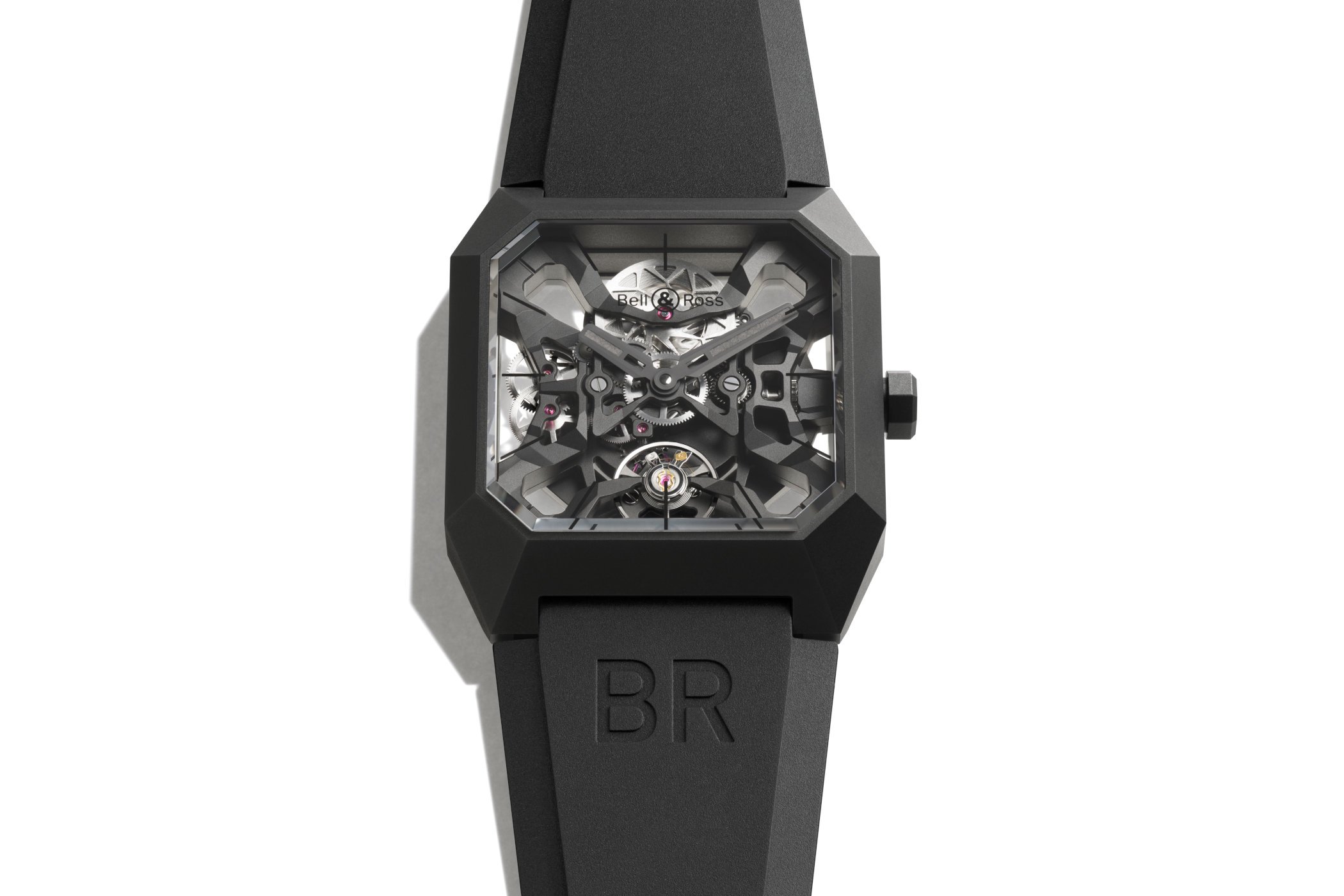This image showcases a remarkably intricate, futuristic-looking watch with a square design characterized by an abundance of straight lines. The entire watch, including both sides of the wristband, is black, giving it a sleek, modern appearance. Inside the watch, visible through the transparent glass face, a complex network of silver gears connects in circular formations. These gears and the interior components contribute to a detailed, mechanical aesthetic.

Prominently featured on the glass at the top of the watch face is the brand name "Bell and Ross," written in black, while the abbreviation "BR" is distinctly etched on the bottom piece of the watch band. The watch hands, blending seamlessly with the intricate gear system, are also black, enhancing the cohesive look. On the right side of the watch is a black winding knob, further contributing to the sophisticated design. The white background of the image makes the watch stand out, with a subtle shadow on the left side adding depth to the overall visual presentation.